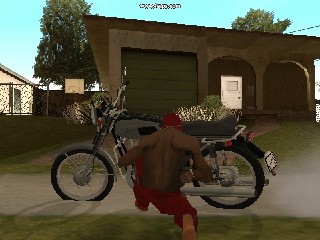The image is a detailed screenshot from a video game, depicting an outdoor scene with a blue sky in the background. Centered in the foreground, a person dressed in gray, with some mentions of red pants and a red hat, is kneeling in front of a gray motorcycle that has a black seat, black wheels, and possibly a basket attached. The motorcycle is positioned with its front facing left and rear to the right. The person kneels partly on a gray sidewalk and partly on grass, focusing their attention on the motorbike.

In the background, a brown building features prominently. To the back right, this building includes a green-doored garage on the left side, two arched openings—one with a white door and another revealing a brown backdrop. Adjacent to the building, and partially obscured by it, are blocky, low-resolution trees. There's mention of a potted plant area containing a bush and white flowers. Additionally, to the building’s left, a fence is visible along with a white structure. Overall, the scene gives off a quaint, suburban feel with simplistic graphics characteristic of a video game environment. Various elements, such as a tall tree and potentially some text at the top of the screen, add further context to the surroundings.